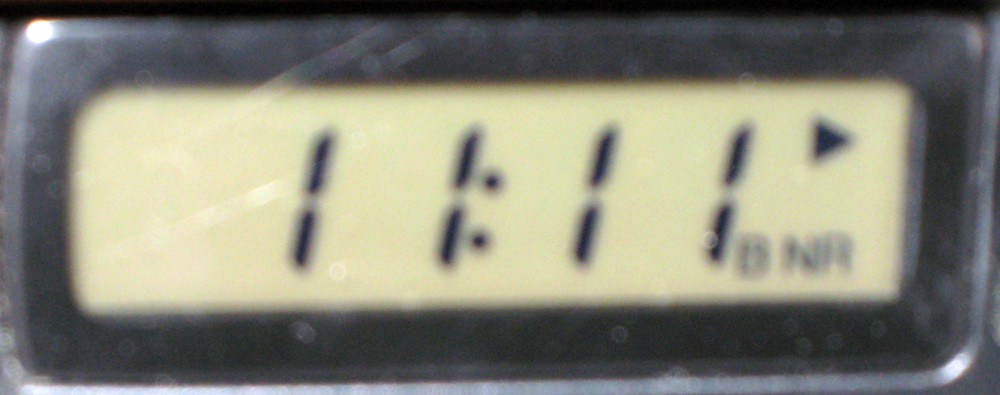This rectangular, horizontally oriented photograph presents a notably blurry image—likely due to either camera shake or outdated technology—of a digital alarm clock. The clock features a black plastic frame with a greenish-white display. Prominently displayed in large black numbers, the time reads "11:11." Additionally, a small triangle icon is visible at the top right corner of the clock face, while some indistinct letters are visible in the bottom right corner. Despite the blurred quality, the clock's essential details, especially the distinct time, are discernible.